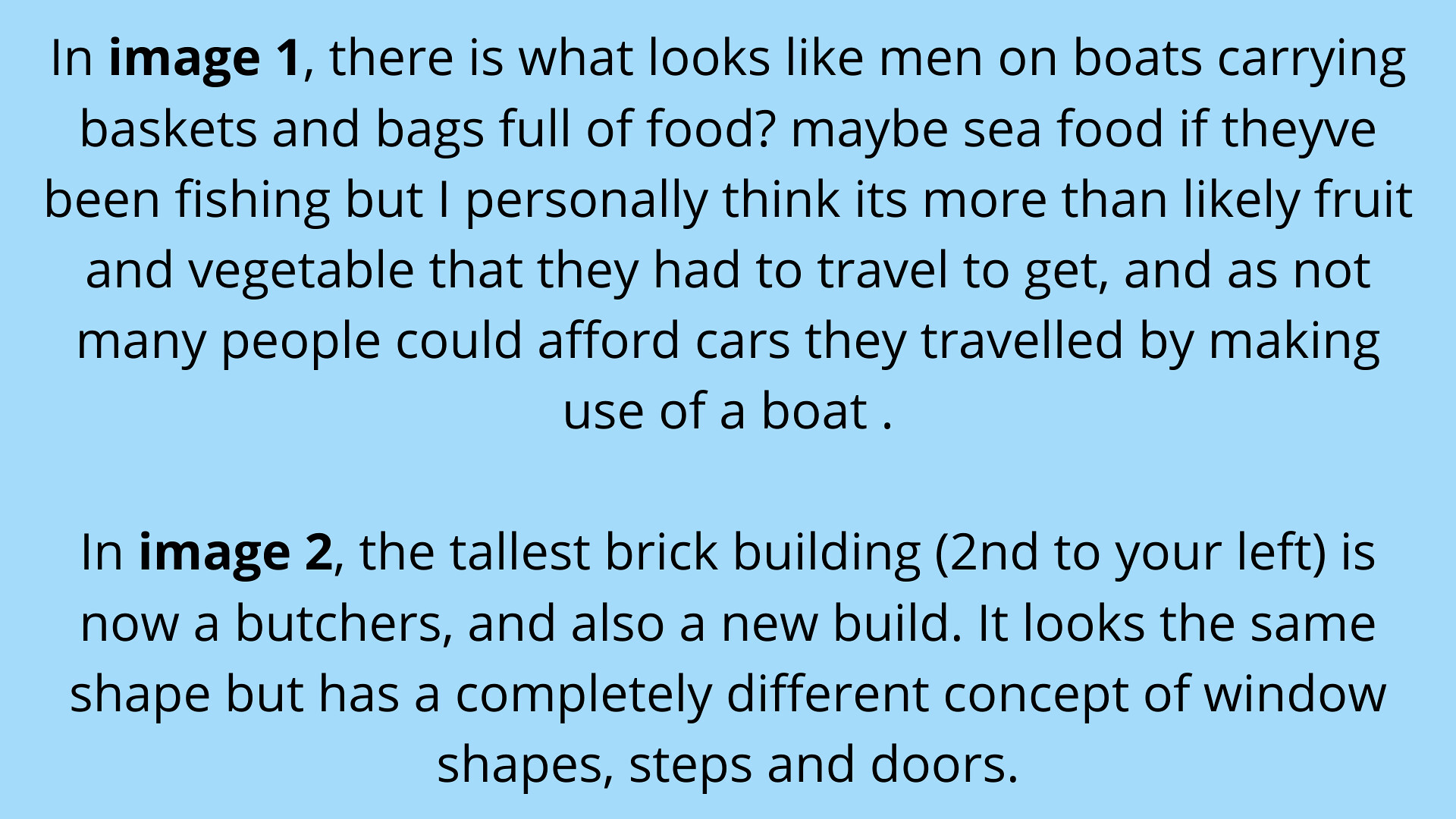The image displays two paragraphs of black text against a light blue background. The first paragraph, with "image one" in bold, describes men on boats carrying baskets and bags full of food, possibly seafood or more likely, fruit and vegetables, which they had to travel to get, given that fewer people could afford cars and thus used boats. The second paragraph, with "image two" in bold, discusses the tallest brick building, specifically the second to the left, which is now a butcher's shop and a new build. While the building retains its shape, it features a completely different concept of window shapes, steps, and doors.